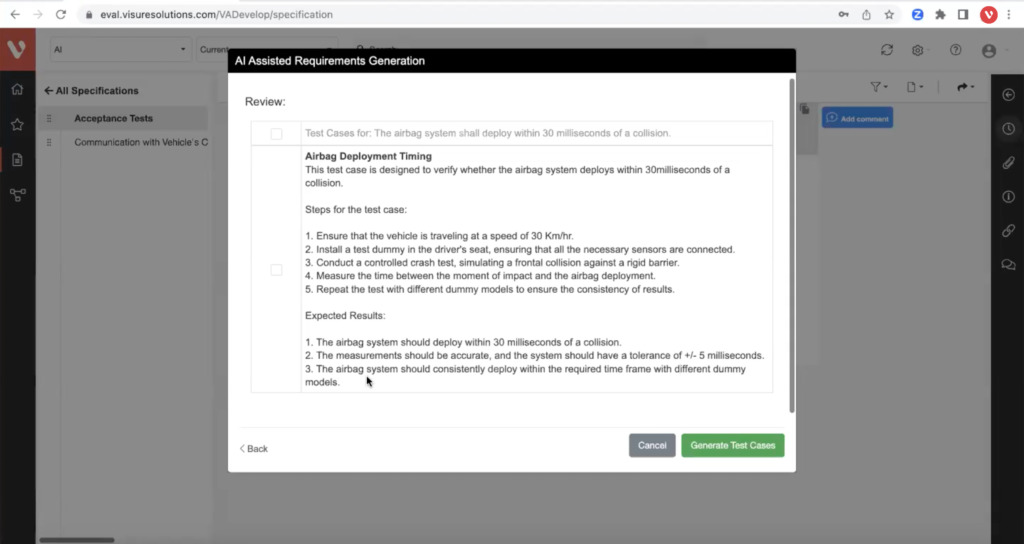Screenshot of the Visor Solutions website focused on AI-assisted airbag system safety testing:

The screenshot captures the webpage from VisorSolutions.com, specifically the product evaluation portal visible through the URL: eval.visorsolutions.com/VA-develop/specification. The browser's URL bar is prominent at the top, with a few options situated on the right-hand side.

Central to the image, the logo of Visor Solutions—a stylized white "V"—is featured twice. On the right, the "V" sits within a red circle, whereas on the left, it appears within a red square that takes on an orange hue due to the greyscale overlay effect applied to the entire screen.

A vertical menu is displayed along the left side of the page, featuring icons for home, starred pages, and potential sharing or linking options that are not entirely clear. Specific sections like "Tests" and "All Specifications" appear as part of a pop-up menu, obscuring much of the underlying content.

The focus of the content is on "AI-assisted requirements generation, review, and test cases for the airbag system." The primary test case outlined is to verify whether the airbag system deploys within 30 milliseconds of a collision. The description provided includes the steps for the test case, listed in five points, and the expected results, detailed in three points.

At the bottom of the pop-up menu, there is link text labeled "Back" in gray. To its right, there is a gray button marked "Cancel," and continuing further right is a longer green button labeled "Generate Test Cases." Overall, the screenshot illustrates simulated testing procedures for a car's airbag deployment system, emphasizing the precision and timing of airbag activation following a collision.